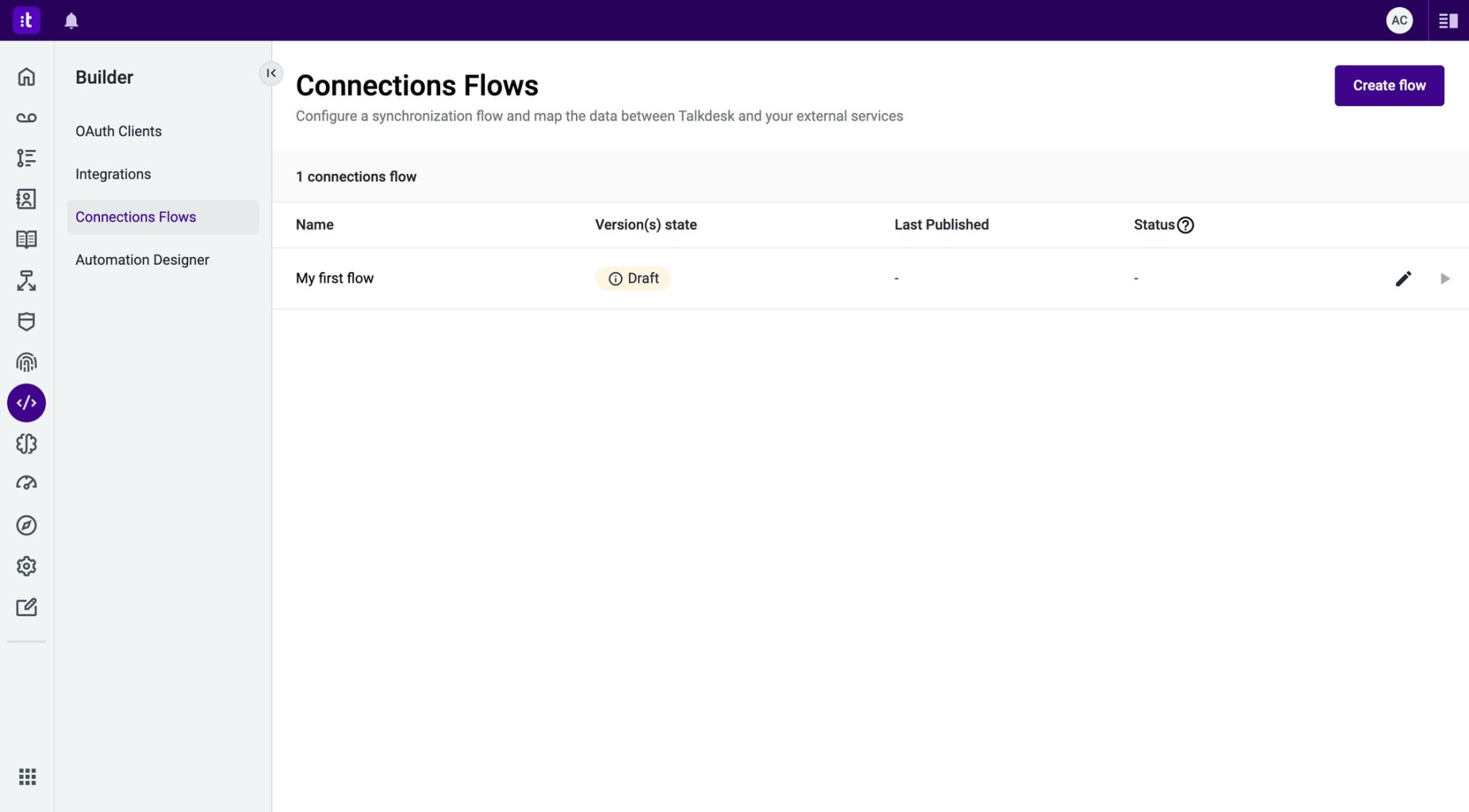Screenshot of a website interface, displaying an internal work screen. The top bar is a deep purple color, featuring a lighter purple circle with the letter 'T' inside it on the right, followed by a bell icon. Adjacent to these is a white circle containing the initials 'AC' and a small rectangle resembling a menu icon.

On the left-hand side is a vertical navigation menu, including items labeled "Builder" represented by a house icon; "Clients" depicted by an upside-down film roll icon; "Integrations;" "Connection Flows" illustrated by a bust image; "Automation Designer" indicated by an open book icon; and various other icons such as a flowchart, shield, and gear, culminating with an icon of a paper and pencil at the bottom.

At the bottom of this sidebar is a square composed of nine smaller squares. The main content area of the screen prominently displays the title "Connection Flows." Below it, a subtitle reads, "Configure a synchronization flow and map the data between Task Desk and your external services." There is a button labeled "Create Flow." A table is shown listing connection flows with columns for "Name," "Version," "State," "Last Published," and "Status." Listed is one entry titled "My First Flow" with a status marked as "Draft."

Overall, the page serves as a configuration interface for managing and mapping data synchronization flows.